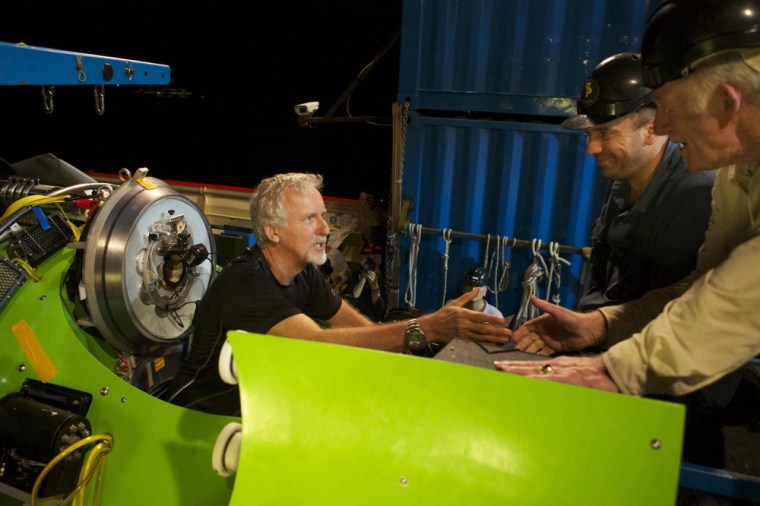In this color landscape photograph, we see a scene involving three Caucasian men centered around a bright neon green pod. The focal point is a famous movie director, known for directing Titanic, who is either entering or exiting the pod. He is a white man with short white hair and a goatee, wearing a black short-sleeved shirt and a black watch on his right wrist. He is seated within the pod, reaching out to shake hands with two other white-haired men. These two men, standing to the right of the image, are wearing black helmets, and both appear to be very happy to engage with the director, as evidenced by their smiles and animated expressions. The pod features a yellow strip of tape and various electronics protruding from the top. The image is taken indoors, with a dark blue background that includes indistinct metal storage units and possibly a security camera or sensor. The bright neon green of the pod prominently contrasts with the otherwise dim surroundings, making for an intriguing and vibrant photograph.